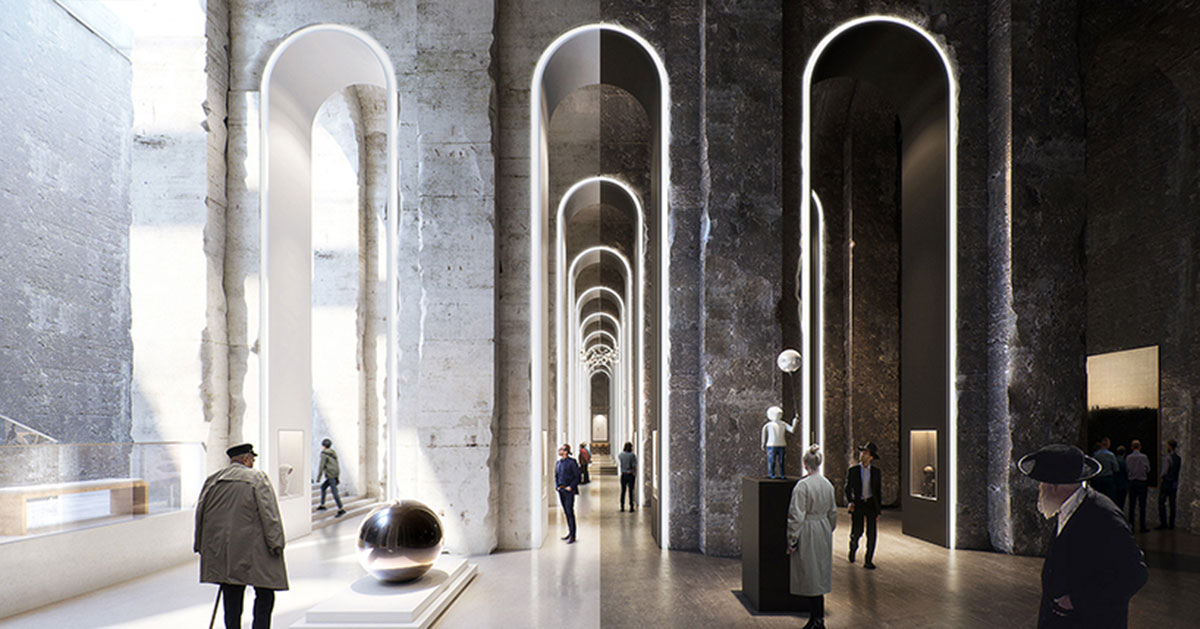This photograph captures a bright and expansive interior of a museum, distinguished by its photorealistic quality. The museum features a series of large arches, each about 25 to 35 feet tall, that form three hallways extending far into the distance. These hallways are constructed with varying shades of marble, with the left in white, the middle in a mix of white and gray, and the right in dark gray marble. The right side of the image showcases a clear glass wall that allows abundant natural sunlight to flood the space, creating a luminous atmosphere.

Scattered throughout the museum are several visitors, both men, and women, dressed in coats. Prominent along the hallway are different art exhibits, including a striking all-silver orb that stands waist-high to an adult, and a statue of a young boy in white except for jean shorts, holding what appears to be a ball or balloon above his head. The arches and hallways are well-lit, adding to the openness of the space. People are seen engaged with these artworks, including two men under the first arch on the left, three men beneath the middle arch, and two men in hats under the third arch, as well as a woman in a trench coat observing the boy statue. Other exhibits and figures, though not as clearly detailed, are also present throughout the visually captivating museum interior.